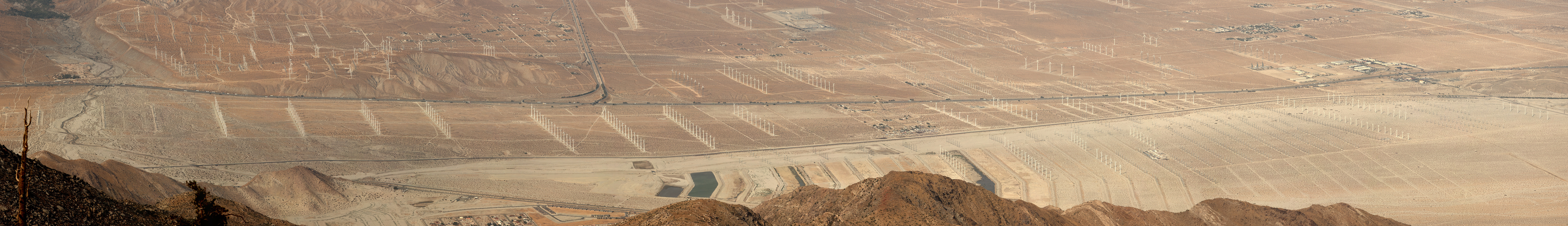A panoramic photograph captures a vast, arid desert landscape, showcasing a stark and expansive terrain. In the foreground, undulating hills and rocky outcrops form a rugged perimeter with a few minute details revealing a complex nestled nearby—possibly a cluster of buildings and some vehicles that are faintly discernible. The barren expanse, devoid of vegetation, stretches endlessly under a beige-hued atmosphere, embodying the stark beauty of the desert. In the distance, slender, linear structures sporadically pierce the horizon, hinting at human intervention. A faint, winding road cuts through the middle of the scene, with minuscule dots suggestive of cars dotting its path. Midway through the picture, indistinct shapes hint at additional man-made formations or encampments, but the true nature remains somewhat ambiguous due to the photo's distant perspective. The overwhelming monotone palette of tans and beiges accentuates the isolation and enormity of this desolate environment.